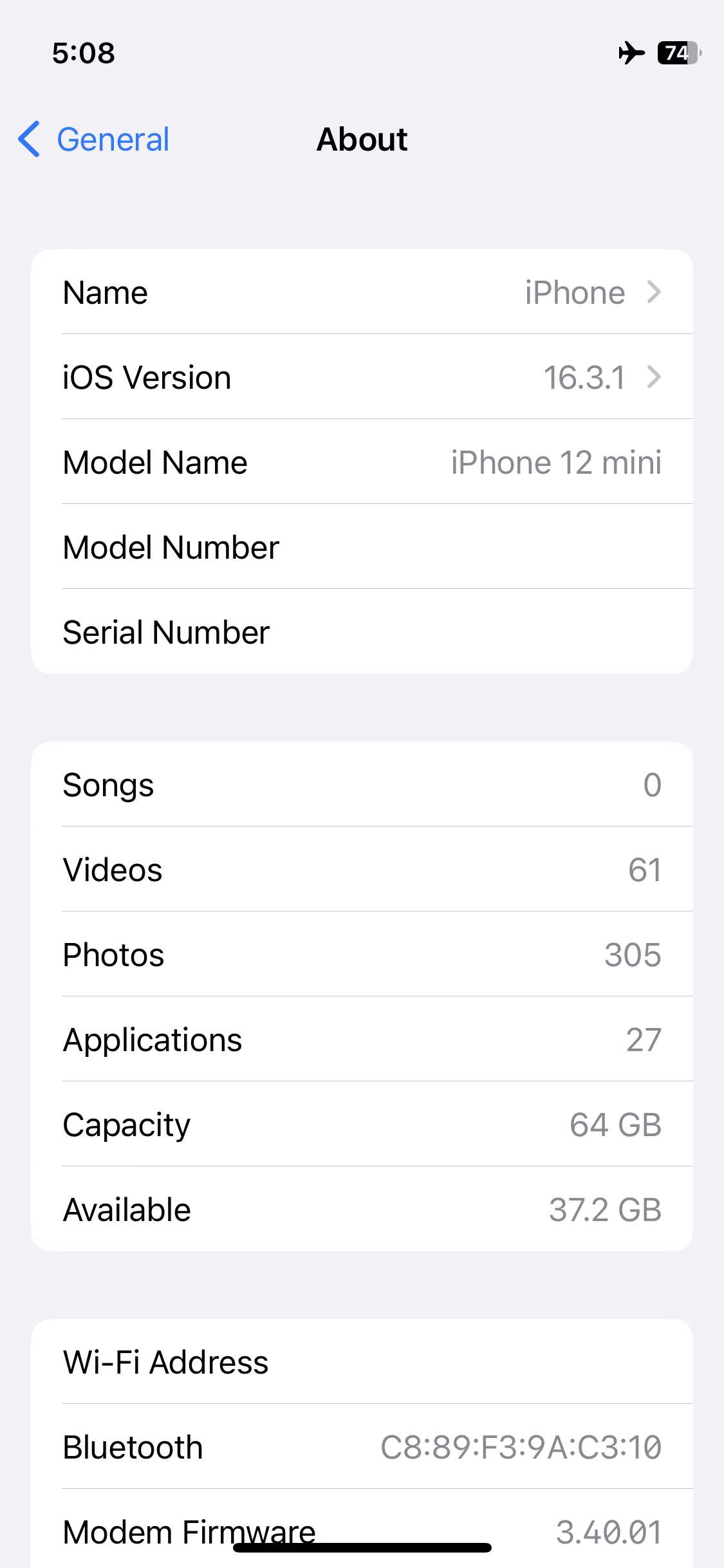A screenshot from a mobile device, possibly a tablet or smartphone, captures a settings page with a dark grey background. The time, indicated in bold black as "508," suggests military time format, given the absence of an AM or PM indicator. On the right-hand side of the status bar, icons for airplane mode and battery level are displayed, with the battery showing as nearly three-quarters full at 74%.

The screenshot features a prominent section header labeled "About," in bold black text, centered on the screen. Below this header is a series of organized sections, each separated by thin grey lines within white rectangles. The first section shows "Name" in black text, likely followed by a user-defined name, which transitions to grey text.

Further down, another section lists detailed information concerning the device's media and storage: 
- Songs: 0
- Videos: 61
- Photos: 305
- Applications: 27
- Capacity: 64 GB
- Available: 37.2 GB

Additionally, another section delineated by some spacing provides network information:
- "Wi-Fi Address" in bold black text, followed by "c8.89.f3.9a.c3.10" in grey.
- "Bluetooth" label likely with its associated Bluetooth address in grey.
- "Modem Firmware" with a black bezel indicating version "3.40.01" on the right-hand side.

This structured and detailed view reveals extensive attributes of the device's settings page, highlighting various technical specifications and storage details.